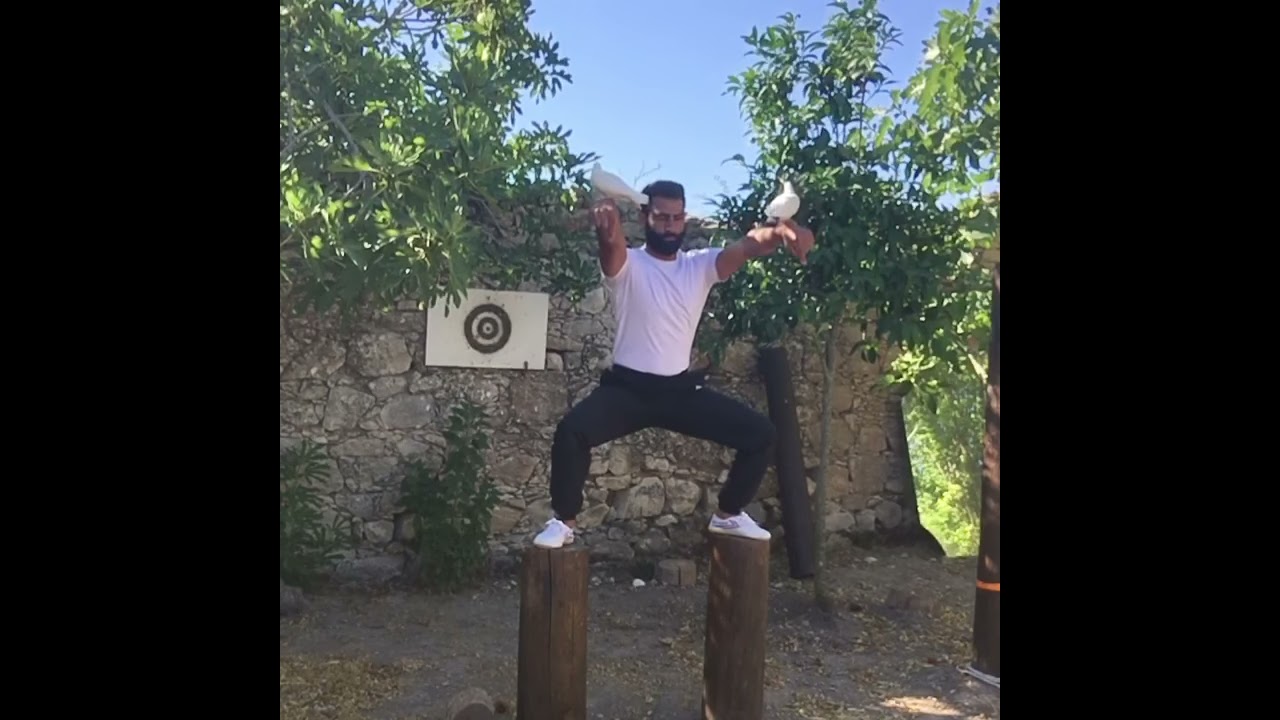In this outdoor scene, a man with dark skin, short black hair, and a black beard stands in a composed horse stance atop two short wooden poles, each foot positioned on a different one. Dressed in a white t-shirt, dark pants, and white sneakers, he faces forward with his knees bent outward and arms extended straight out in front of him, where a white dove gracefully perches on each arm. The backdrop features an old stone wall made of variously sized square and rectangular stones, adorned with overgrown vegetation such as shrubs and what appear to be olive trees. Below the poles, the ground is scattered with dirt and leaves. Prominently displayed on the wall is a target painted on a piece of white wood, suggesting a space used for target practice. The scene is set under a clear blue sky, adding to the serene but disciplined ambiance of the image.